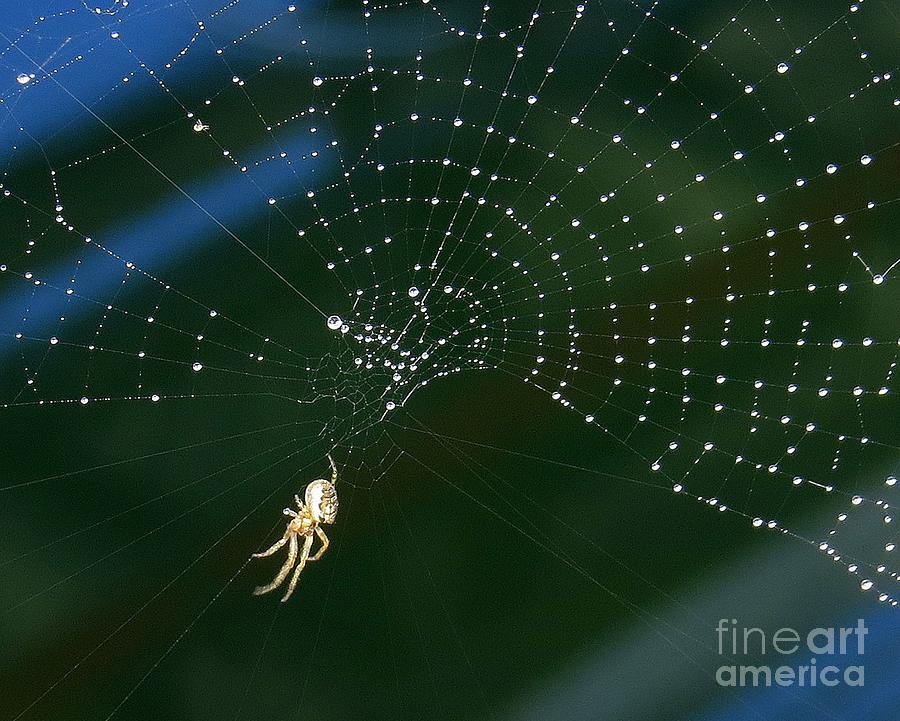This horizontal rectangular image is a detailed, artist's illustration of a spider web with a spider hanging from it. Set against a black background that includes subtle blue shading in the corners, the web stretches across the top of the frame. The junctions where the vertical and horizontal threads of the web meet are illuminated, creating intricate, lighted patterns. The web's center is notably complex, featuring many small, glowing circles. Seemingly caught in mid-construction, the web has a portion at the bottom that remains unfinished.

The spider, prominently showcased against the dark backdrop, is predominantly white with hints of brown and yellow on its round abdomen and legs. Its legs, colored in yellowish-white hues, are visible as it appears to be in the act of weaving. The spider’s form is vivid and detailed, almost suggesting a human-like facial quality.

Scattered throughout the web, particularly at the various connecting points, are numerous glistening water droplets, adding to the ethereal quality of the image. The composition also features a black oval shape dominating much of the background, enhancing the visual contrast. Finally, a watermark in gray text that reads "Fine Art America" is located in the lower right corner, indicating the source and potential availability for purchase.